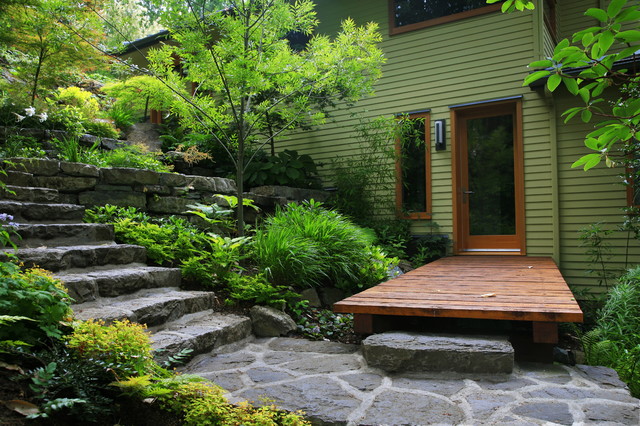This image captures the lush and meticulously maintained backyard of a light green house with contrasting dark brown trim. The scene is centered around the house's back entrance, which features a dark brown, partially glass door paired with a tall, slender window. Just outside the door, a small wooden deck, also brown, extends to meet a stone-paved walkway. On the left side of the image, a set of gray stone stairs ascends to a charming porch area. The entire yard is enveloped in verdant greenery, with vibrant shrubs and trees flourishing around the house, casting generous shade and adding to the serene ambiance. Notable for its well-kept appearance, the backyard suggests a peaceful, inviting outdoor space, ideal for relaxation and enjoyment.